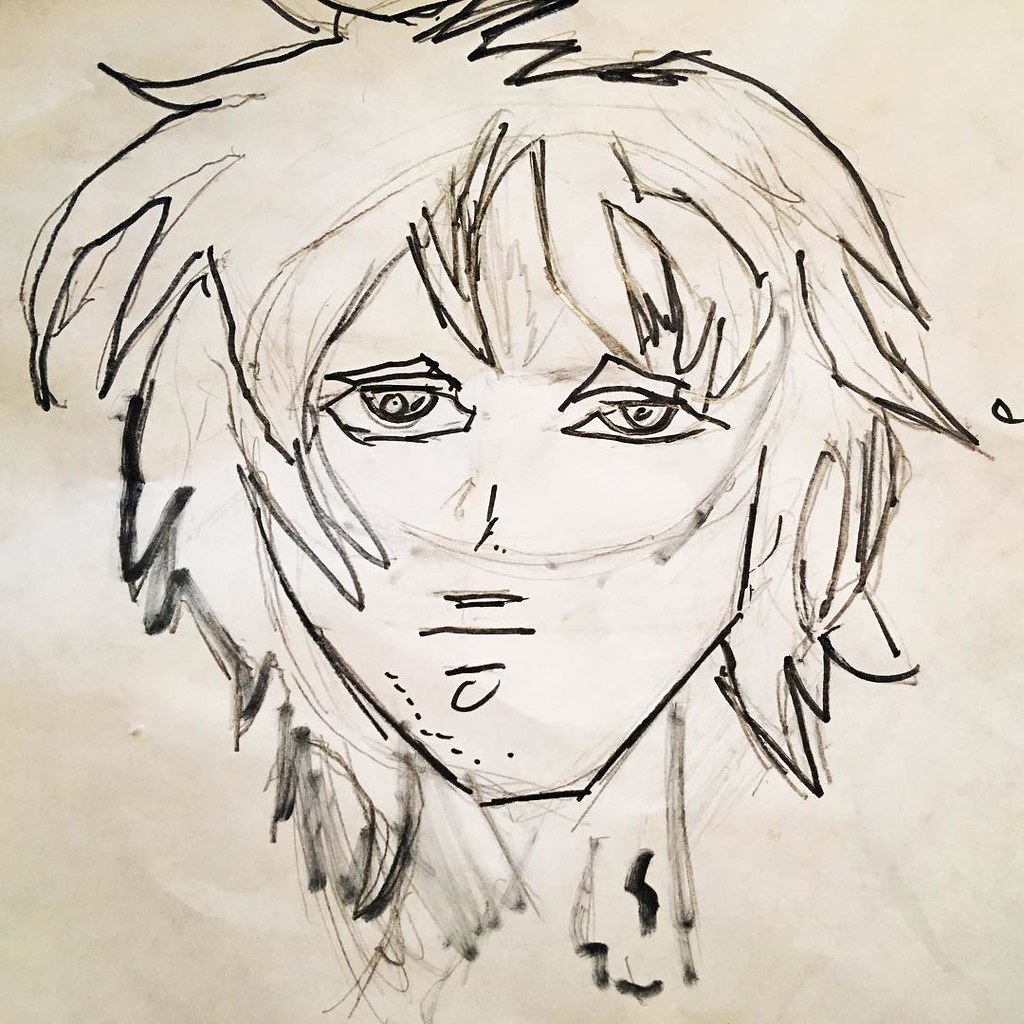The image is a pencil sketch of a man's head and neck, rendered in a comic book style with exaggerated features and rough lines. The man's chin is sharply angular, drawn with three distinct lines, while the sides of his head are sketched with two lines each. His eyes are large and angular, adding to the comic-like appearance. The man's hair is messy, extending just past his ears and is sketchy in its representation, suggesting a 'bedhead' look. Dot markings and a small curly line adorn his chin, which contributes to the rough texture of the drawing.

The man's expression is rather dull and emotionless, with a hint of sadness in his eyes, enhancing the overall enigmatic atmosphere. One eye appears misaligned, possibly a lazy eye, with a strange circular marking around it. The sketch has an unfinished, learning-practice quality, indicating the artist might be still honing their skills. It's mostly shaded with a pencil, with some areas possibly highlighted using marker or watercolor paint, which adds depth and contrast. The entire artwork appears to be digitally scanned, as suggested by the texture and coloration, reflecting a clean, digital upload rather than a photograph.